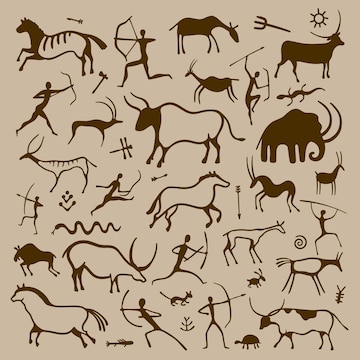This is a square image with a light brown, ecru-like background, depicting what appears to be ancient cave drawings. The objects are illustrated in a very dark brown, simplistic style, akin to hieroglyphics or vector art imitating such. Among the various images, one can see stick-figure hunters in dynamic poses: some are shooting bows and arrows, some running with their weapons at their sides, while others hold staffs or hatchets above their heads. The game being hunted includes a diverse array of animals, such as horses, cows with horns, deer, and even a mammoth resembling an okapi. Smaller creatures like snakes, beetles, dragonflies, a rabbit, a turtle, and fish are also present. A prominent sun occupies the upper right corner of the image, overseeing the entire scene.